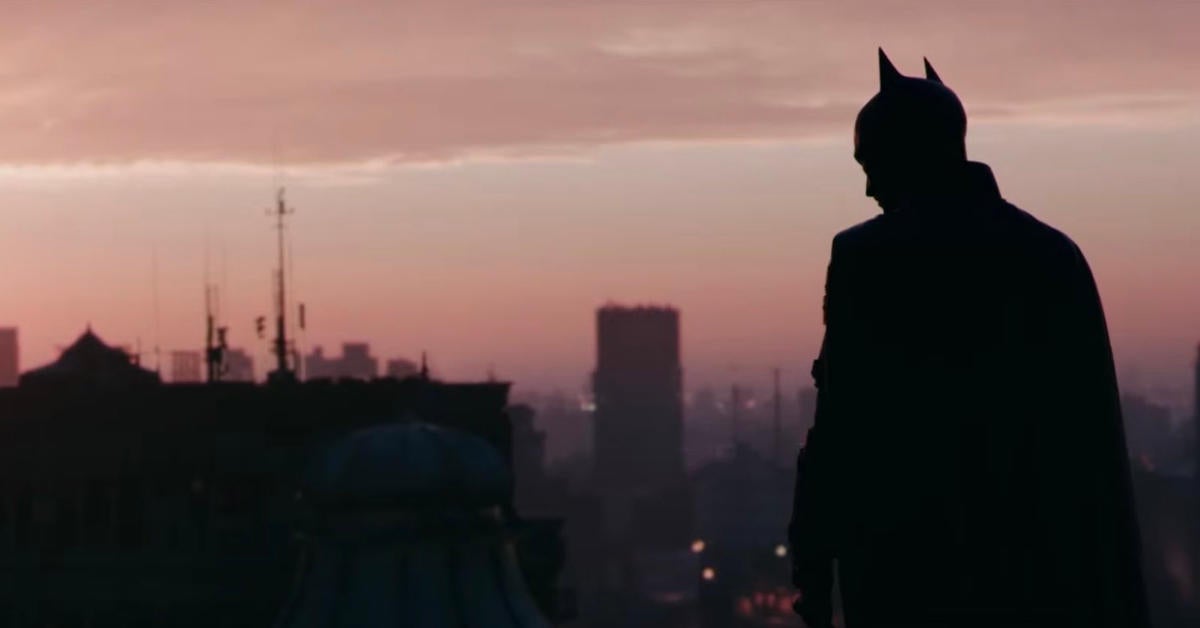The scene appears to be a dramatic moment from a Batman movie, characterized by a nighttime atmosphere with a purplish background that gradates from a dull, greasy gray to orange near the horizon. At the center is the silhouette of Batman, his back turned to the viewer, head slightly bowed as if in deep contemplation, with his iconic ears and cape prominently visible. The sky above is dark, streaked with red and purplish clouds, contributing to the moody ambiance. Scattered about are blurry silhouettes of buildings and telephone poles, some with small lights twinkling in distant windows. Wiring and water tanks are noticeable details among the rooftops, adding to the gritty urban landscape. On the left, a particularly tall building with an antenna stands out against the fuzzy skyline. Batman appears to be on a rooftop, level with other tall structures in this somber, dusk-to-evening setting, his masked visage partially revealing the left profile of his face as he gazes down upon the city.